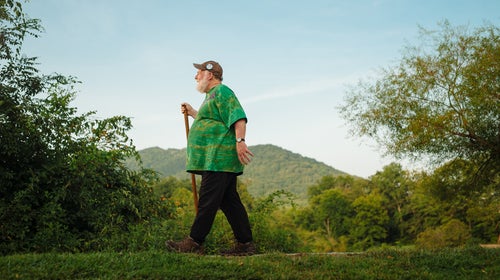In this outdoor photograph, an older man with a distinctive white beard, resembling a shorter Santa Claus beard, is captured in profile as he walks from right to left along a grassy trail. He's equipped with a brown wooden walking stick in his right hand, and wears a brown baseball hat adorned with a pin, along with a green shirt featuring light green accents. His outfit includes black or navy cotton pants, brown hiking boots, and a watch with a black band on his left wrist. The man, who has a larger belly and thinner legs, is positioned against a backdrop of a green, tree-covered mountain that rises beneath a blue sky dotted with light clouds. Surrounding him in the foreground are various shrubs and bushes, suggesting a verdant, natural setting typical of a spring or summer day. The man appears to be enjoying a solitary hike in this serene, lush landscape.